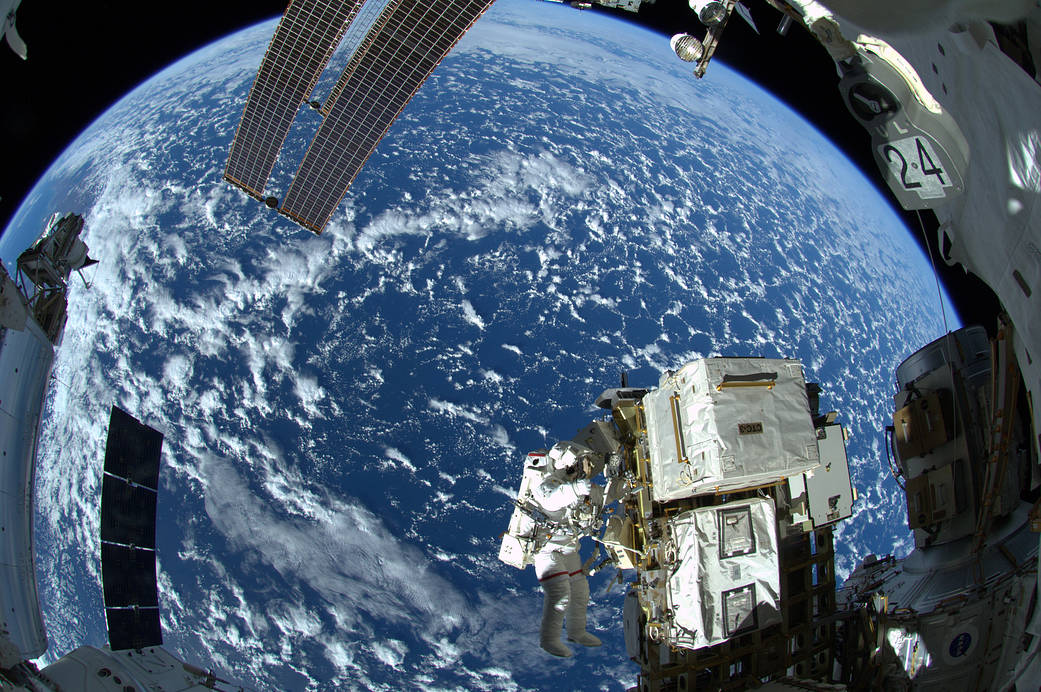In this captivating photograph, an astronaut is seen diligently working outside the space station, fully adorned in a complete astronaut suit. He is floating gracefully in the microgravity environment while securely gripping a handle attached to an intricate arrangement of equipment boxes, all meticulously organized and fastened to a central platform. The image, apparently captured from within the space station, showcases a breathtaking view of Earth in the backdrop, with vast expanses of blue oceans and swirling white clouds. Sunlight floods the scene, illuminating the astronaut and his gear with a vivid, radiant glow, while casting portions of his form in contrasting shadow, adding depth and drama to the composition.